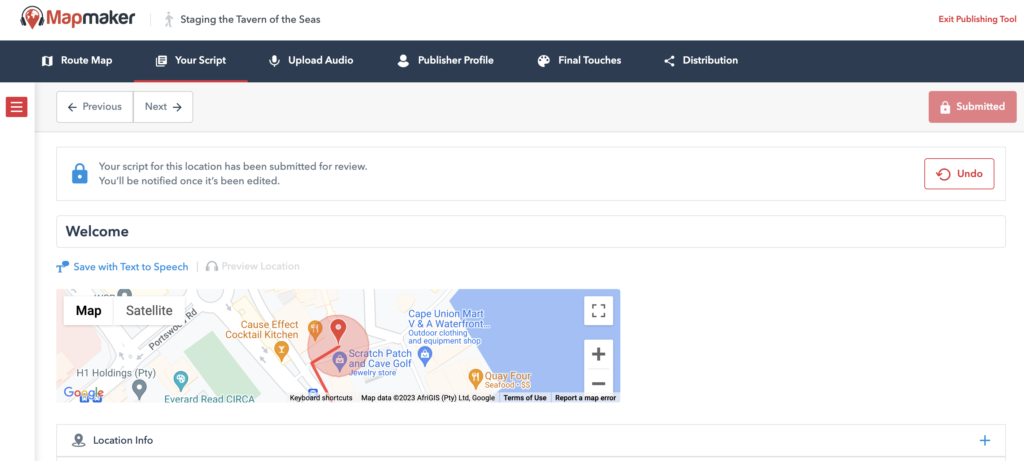This screenshot from MapMaker features the "Tavern of the Seas" staging area. At the top, a blue banner runs beneath the word "MapMaker," displaying navigation options such as Route Map, Your Script, Upload Audio, Publisher Profile, Final Touches, and Distribution, all in white text. Below this banner, three boxes are aligned: a small red one showing a three-line menu icon, and two buttons labeled Previous and Next. Additionally, there is a slightly discolored red button labeled "Submitted" on the right-hand side, indicating submission status.

Proceeding downward, the screen reads, "Your Script for this location has been submitted for review. You will be notified once it has been edited," accompanied by a red Undo button on the far right. Beneath this message is the word "Welcome." 

Following this, a map graphic is displayed, highlighting points of interest such as the Cause Effect Cocktail Kitchen, the Scratch Patch and Cave Golf, and Cape Union Mart V and a Waterfront. The map is sourced from Google Maps but lacks specific location identifiers. Below the map, grey text reads "Location Info" next to a plus button on the right-hand side.